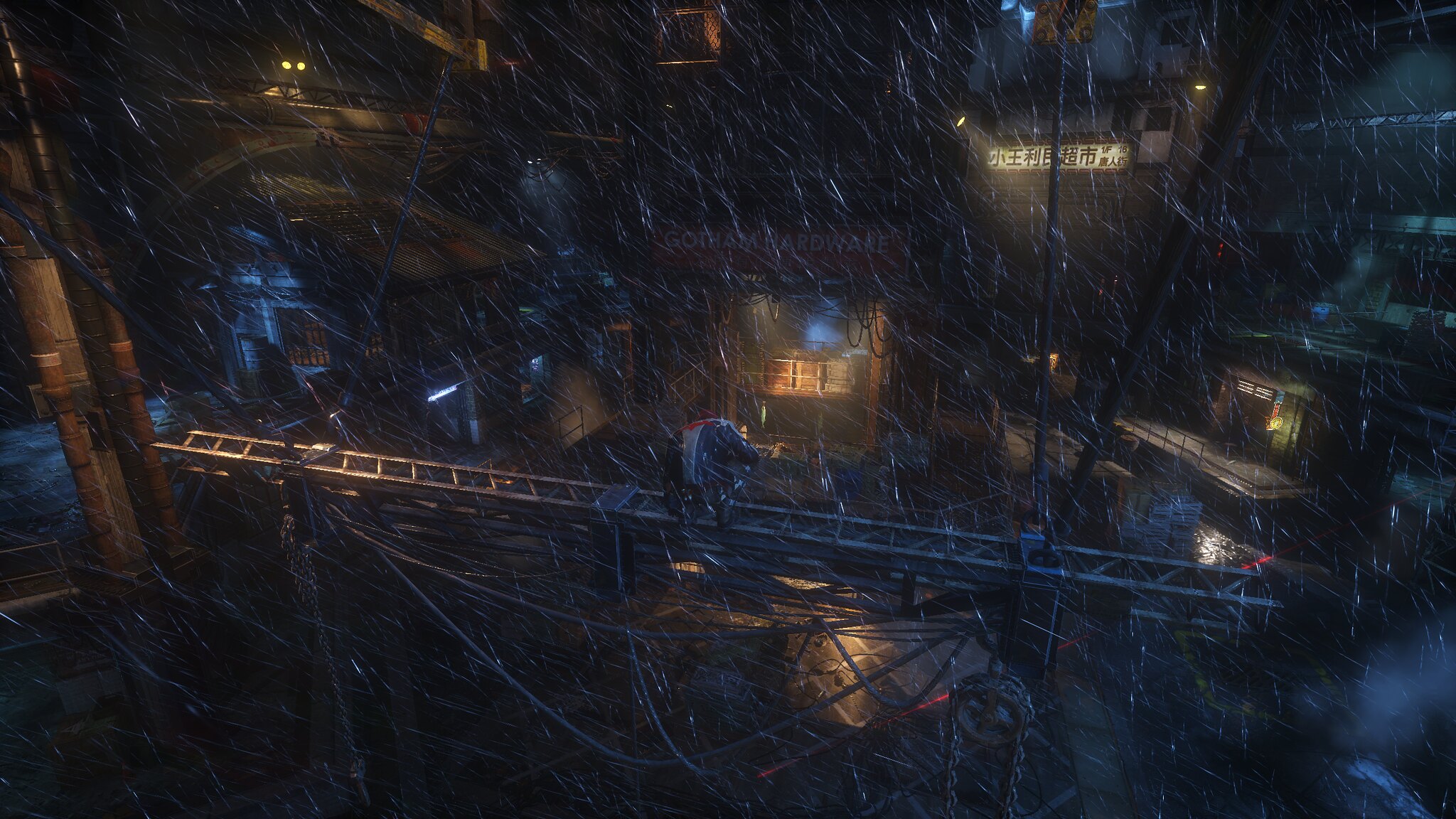This captivating image is a piece of digital art illustrating a dark and rainy urban scene. The industrial-looking cityscape is cloaked in shadows, with a multitude of buildings encircling the area and minimal lighting. At the center, a long structure that resembles a ladder extends horizontally from the left to the right, draped with tangled wires and cables. The darkness makes it challenging to discern the figure moving across this ladder-like structure—it's ambiguous whether it is a person or an animal. On the left side of the image, telephone poles with additional wires contribute to the intricacy. Among the dense arrangement of elements, one visibly illuminated storefront features a sign with Chinese characters. The subtle play of lights from buildings casts hues of red, blue, yellow, and white against a backdrop dominated by shades of grey and brown, adding to the scene's mysterious and somber atmosphere.